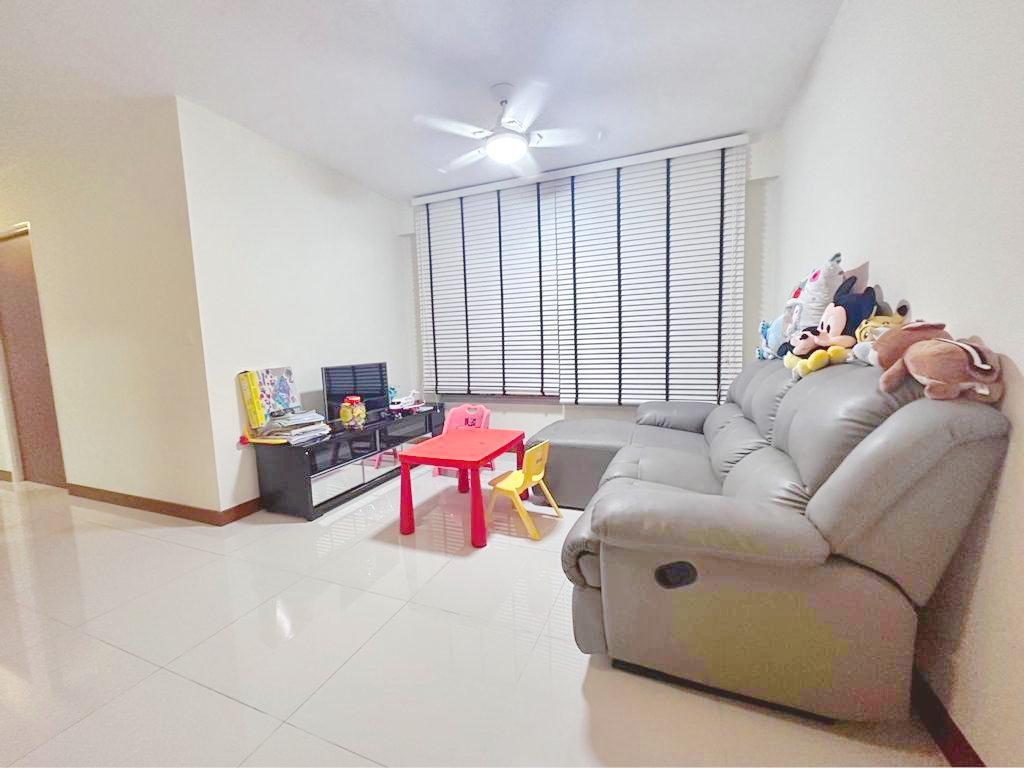The image showcases a cozy room with a white ceiling and off-white, almost beige walls. On the right side of the room, there's a plush grey couch adorned with several stuffed animals, including a prominent Mickey Mouse head in the center and a brown stuffed animal lying on its stomach. The floor is covered with off-white, flat tiles. A small yellow and pink chair is positioned next to a tiny red table, creating a cheerful play area. Nearby, a black table holds a collection of small books, which appear to be coloring books, along with some board games. To the right, white and black-lined blinds hang over a window, partially obscured. Above, a combination light and ceiling fan fixture is installed. Down a visible hallway, there is a brown door. Additionally, a brown baseboard trim runs along the base of the walls, blending into the flooring.